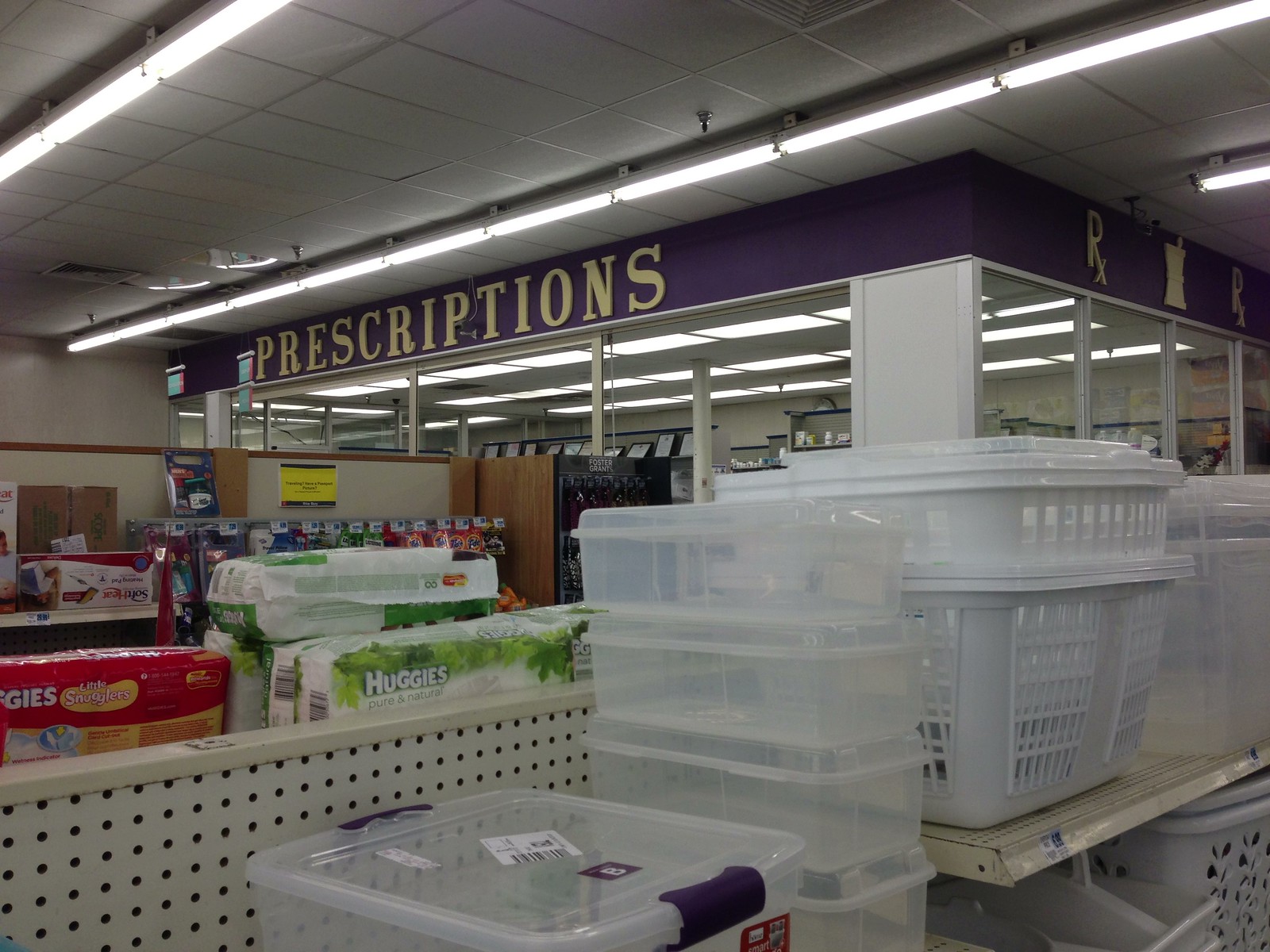The image depicts the inside of a convenience store with a prominent pharmacy section. In the foreground, a variety of storage boxes and clear plastic totes with purple handles are displayed on pegboard aisles. To the side, white slatted laundry bins stand on shelves. Further along, Huggies diapers in distinctive red and white packages are visible on the next aisle. Beyond the diaper section, shelves possibly holding razor blades can be seen. The pharmacy area is prominently marked by a purple-topped structure with glass walls, labeled 'prescriptions' in yellowish letters. Fluorescent lighting tracks run throughout the image, with one positioned directly in front of the prescription sign and another in the top right corner, illuminating the store's numerous shelves and products.